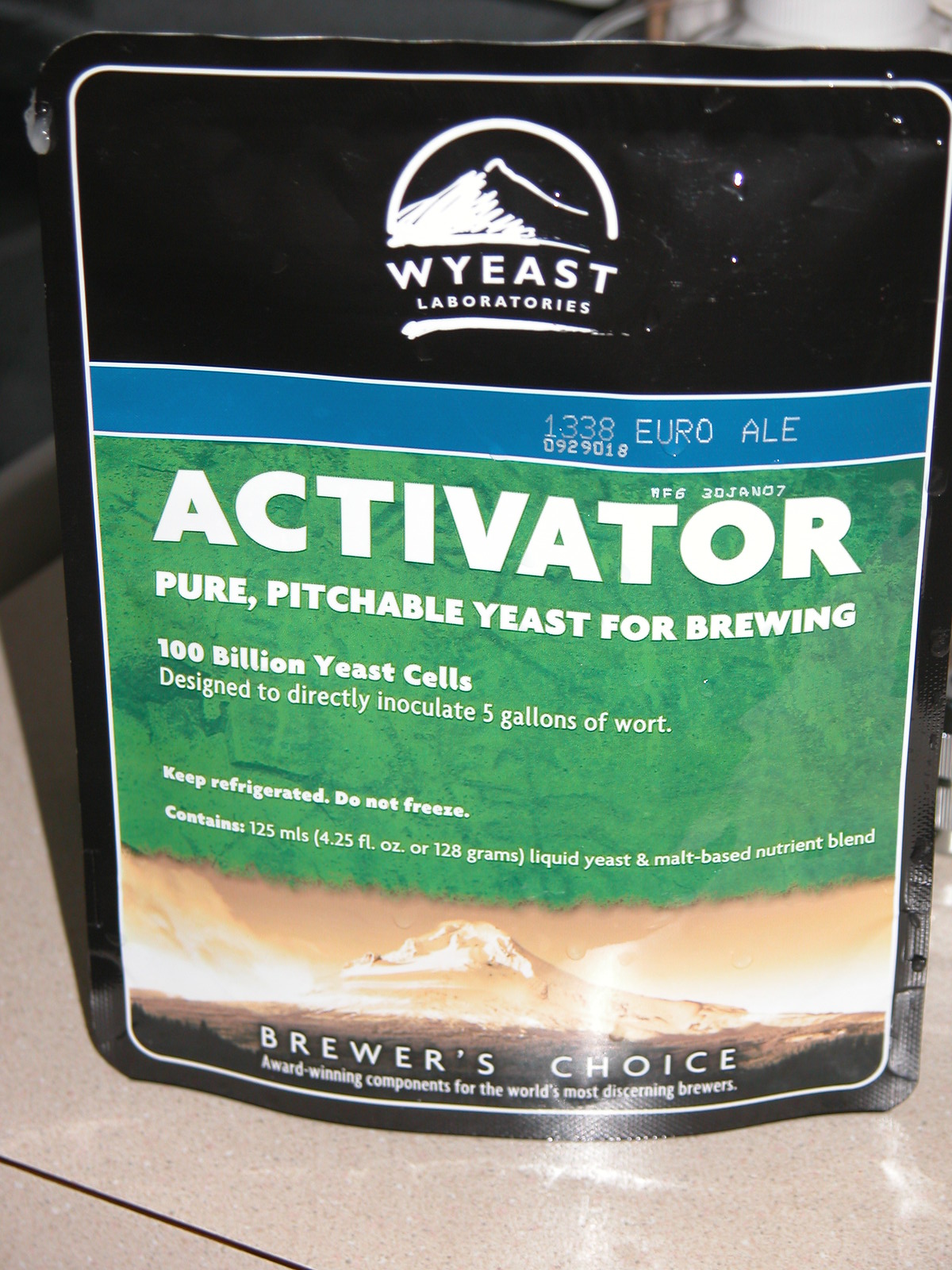This indoor photograph captures a vertically rectangular, black plastic package set against a kitchen backdrop with a beige countertop, black trim, and a black backsplash wall. The package features a prominent black top with a mountain logo and text reading "WY East Laboratories," beneath which a blue band specifies "1339-092-9018 Euro Ale" in white letters. Below this, a green section with white text details the product as "Activator, pure pitchable yeast for brewing, 100 billion yeast cells designed to directly inoculate five gallons of wort. Keep refrigerated, do not freeze. Contains 125 mLs (4.25 fluid ounces) of 128 grams liquid yeast and malt-based nutrient blend," dated "20th January 07." At the bottom of the package, a sepia-toned graphic of a mountain is accompanied by the phrase "Brewer's Choice, award-winning components for the world's most discerning brewers." The package is designed to stand upright by itself, enhancing its distinctive and professional presentation.